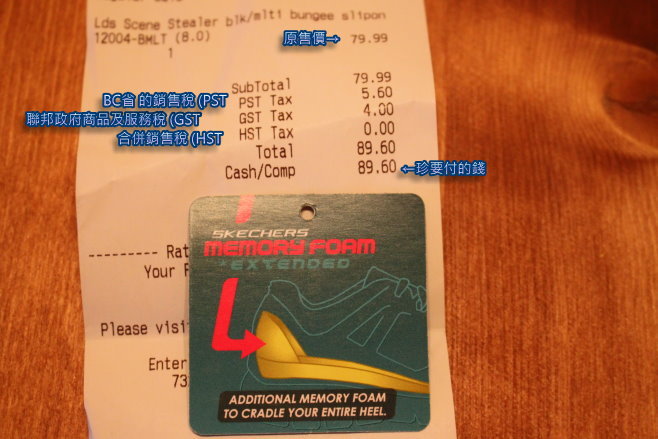A close-up image of a receipt details the purchase of an item listed as "LDS Scene Stealer Black/Multiple Bungee Apron" priced at $79.99. The receipt, primarily displayed in English, shows a subtotal of $79.99 and two separate tax entries of $5.60 and $4.00, summing up to a total amount of $89.60. This total payment is labeled as "Cash/Comp $89.60." Chinese characters are prominently featured around the receipt, with a set of blue Chinese letters and an arrow pointing at the total amount of $89.60 on the right-hand side and additional blue Chinese characters around the tax entries on the left. At the bottom portion of the image, a piece of cardboard sticker is partially covering the receipt, detailing "Skechers Memory Foam Extended." The information highlights the added comfort feature of extended memory foam designed to cradle the entire heel. This description is explicitly noted in English, and the memory foam feature is emphasized. The Chinese characters might be indicative of either manufacturing details or added context possibly signifying that the products are made in China.